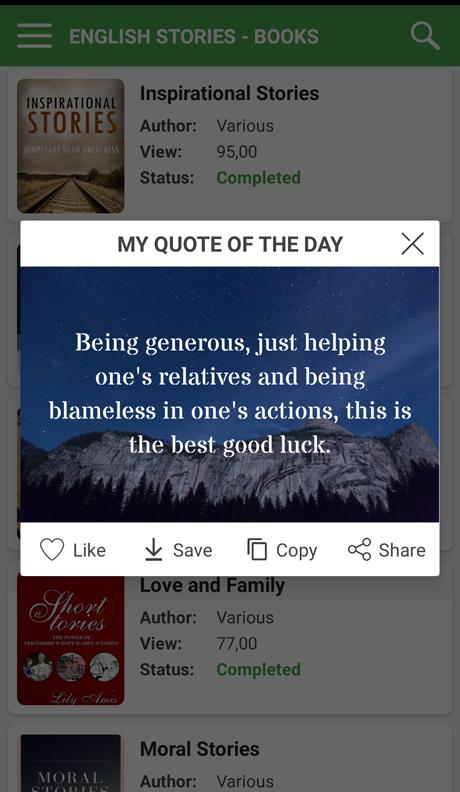In this cellphone screenshot, the viewer's screen displays an English stories webpage with various story categories visible in the background, albeit slightly blurred and grayed out. At the very top of the webpage, the category titled "Inspirational Stories" is clearly visible. Further down, other categories like "Love and Family" and "Moral Stories" can be made out towards the bottom of the screen. 

In the middle of the screen, there is a prominent rectangular pop-up that captures most of the viewer's attention. This pop-up window is significantly brighter than the underlying webpage, making the background details less distinct. The header of this pop-up reads "MY QUOTE OF THE DAY" in bold, all-capital letters. There's a clickable 'X' icon in the top-right corner of the pop-up for closing it.

The background image within the pop-up depicts a serene nighttime scene of mountains and trees silhouetted against a dark, navy blue sky. The quote displayed within the pop-up states, "Being generous, just helping one's relatives, and being blameless in one's actions – this is the best good luck." Below the quote, there are icons for heart (likely for favoriting), save, copy, and share options, suggesting interactive features for the user to engage with the quote.